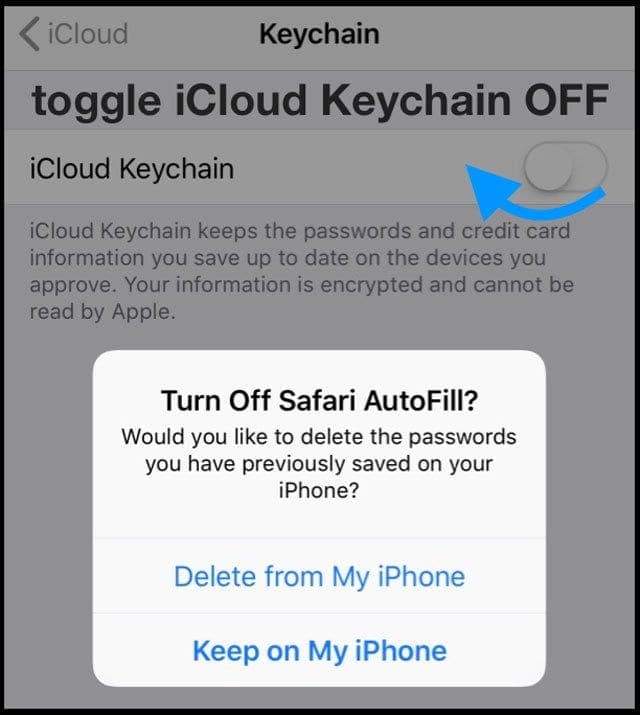This screenshot displays the iCloud Keychain settings interface, characterized by a gradient of gray shades forming the background. At the top-left corner, a gray, triangle-shaped back arrow points to the left, flanked by the word "iCloud" in muted gray.

The central focus is the word "Keychain" in bold black. Beneath this, a darker gray bar features the label "Toggle iCloud Keychain Off". Below this, on a lighter gray bar, the phrase "iCloud Keychain" is accompanied by a toggle button currently set to the off position, which can be slid to the right to activate it. Directly below, a blue arrow curves clockwise, suggesting a refresh action.

A paragraph of text clarifies the function and security of iCloud Keychain: "iCloud Keychain keeps the passwords and credit card information you save up to date on the devices you approve. Your information is encrypted and cannot be read by Apple."

Central to the interface, a white dialog box prominently asks, "Turn off Safari Autofill?" followed by the question, "Would you like to delete the passwords you have previously saved on your iPhone?" Below this query, two blue-button options are presented: "Delete from my iPhone" and the bolded "Keep on my iPhone".